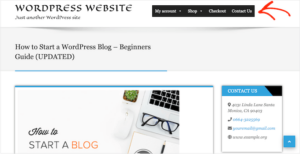This image is a partial screenshot of a WordPress website, rectangular in shape and oriented horizontally on the screen. In the upper left corner, the text reads "WordPress website. Just another WordPress site." To the right, a black navigation bar features options including "My Account," "Shop," "Checkout," and "Contact Us." At the far upper-right corner, an arched-shaped arrow points inward towards the black navigation bar.

Central to the screenshot, a prominent gray banner spans across the page, displaying the text "How to Start a WordPress Blog: Beginner's Guide Updated." Below this banner is a blue line, followed by a white background. This section contains two boxes: one titled "How to Start a Blog," and another titled "Contact Us." The "Contact Us" box features a blue banner at its top, with a small black section on the upper right side of the box.